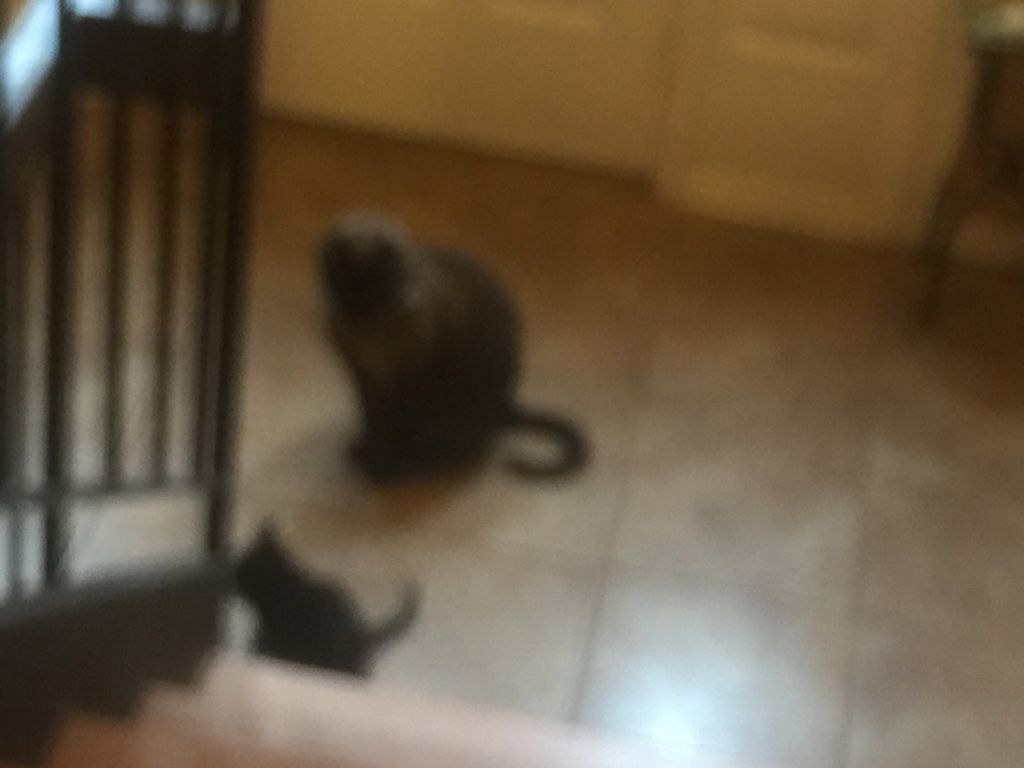A very blurry color photograph captures a tender moment on a brown tiled floor with large tiles and darker grout. In the center of the image, a dark brown and black cat sits, its tail outstretched and curling gracefully along the floor. The cat's gaze is fixed downward at a tiny black kitten positioned nearby. On the left side of the frame, a descending staircase with a dark-colored handrail adds a sense of depth and structure to the scene. In the blurred background, a white wall and the lower portion of a white door are visible, along with the edge of a brown table on the right side of the image. Though the photo lacks clarity, the composition reveals a cozy, domestic setting, highlighting the interaction between the two felines.